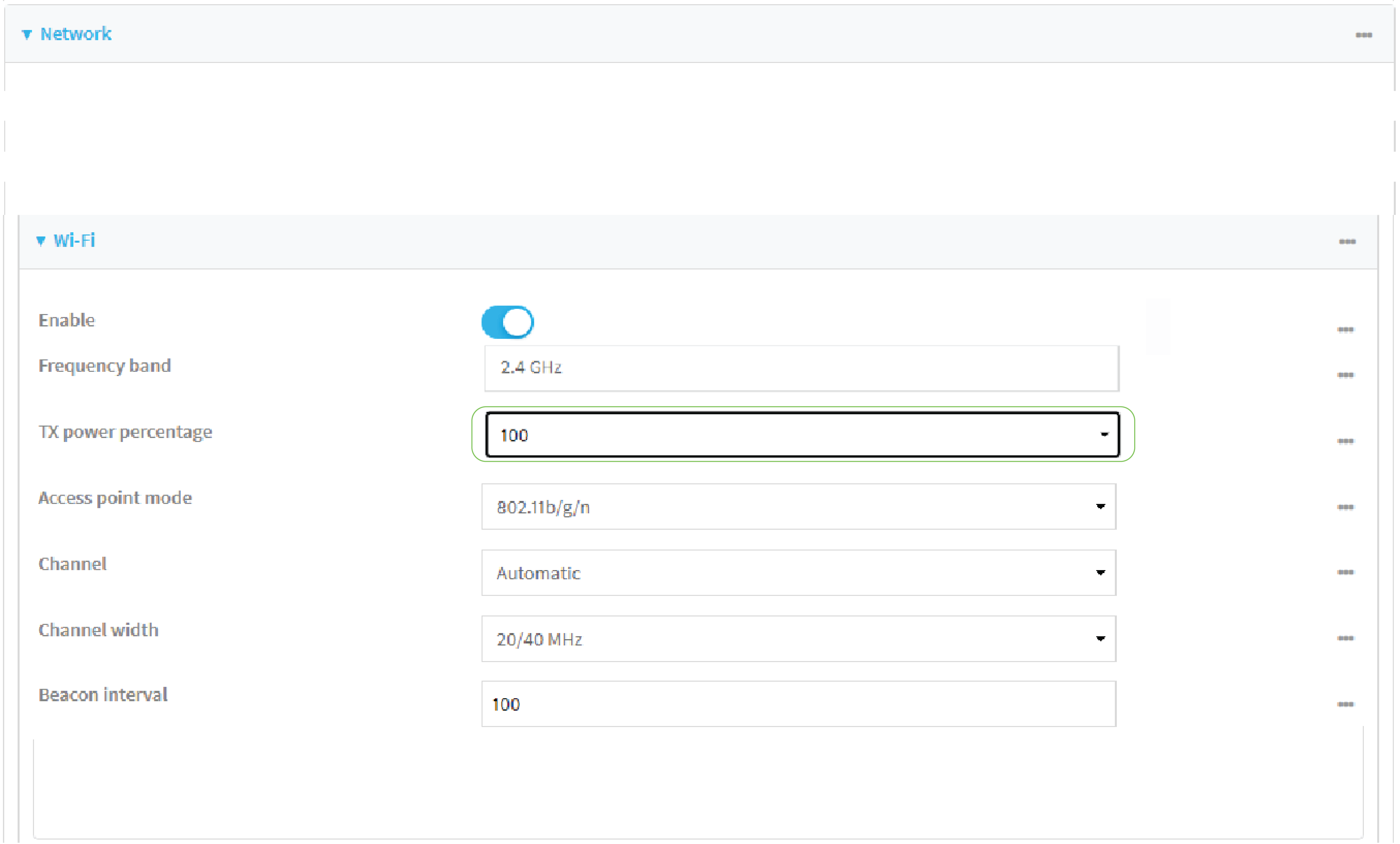The image displays a user interface screen set against a white background, showcasing various Wi-Fi network settings in blue text. At the top, there is a heading labeled "Network" in blue. Below that, a section titled "Wi-Fi" is also highlighted in blue. 

An "Enable" option is shown, accompanied by a toggle switch that is currently active, indicated by its shaded blue color with a white circle. The frequency band is listed as "2.4 GHz" (with "G" and "H" in uppercase), and the transmission power (TX Power) is set to 100%.

The interface also includes information about the access point mode, specified as "802.11b/g/n." The channel setting is on automatic, and the channel width is specified as "20/40 Hz." The beacon interval is set to 100 milliseconds. To the far right of each setting option, there are three vertical dots indicating additional menu options.